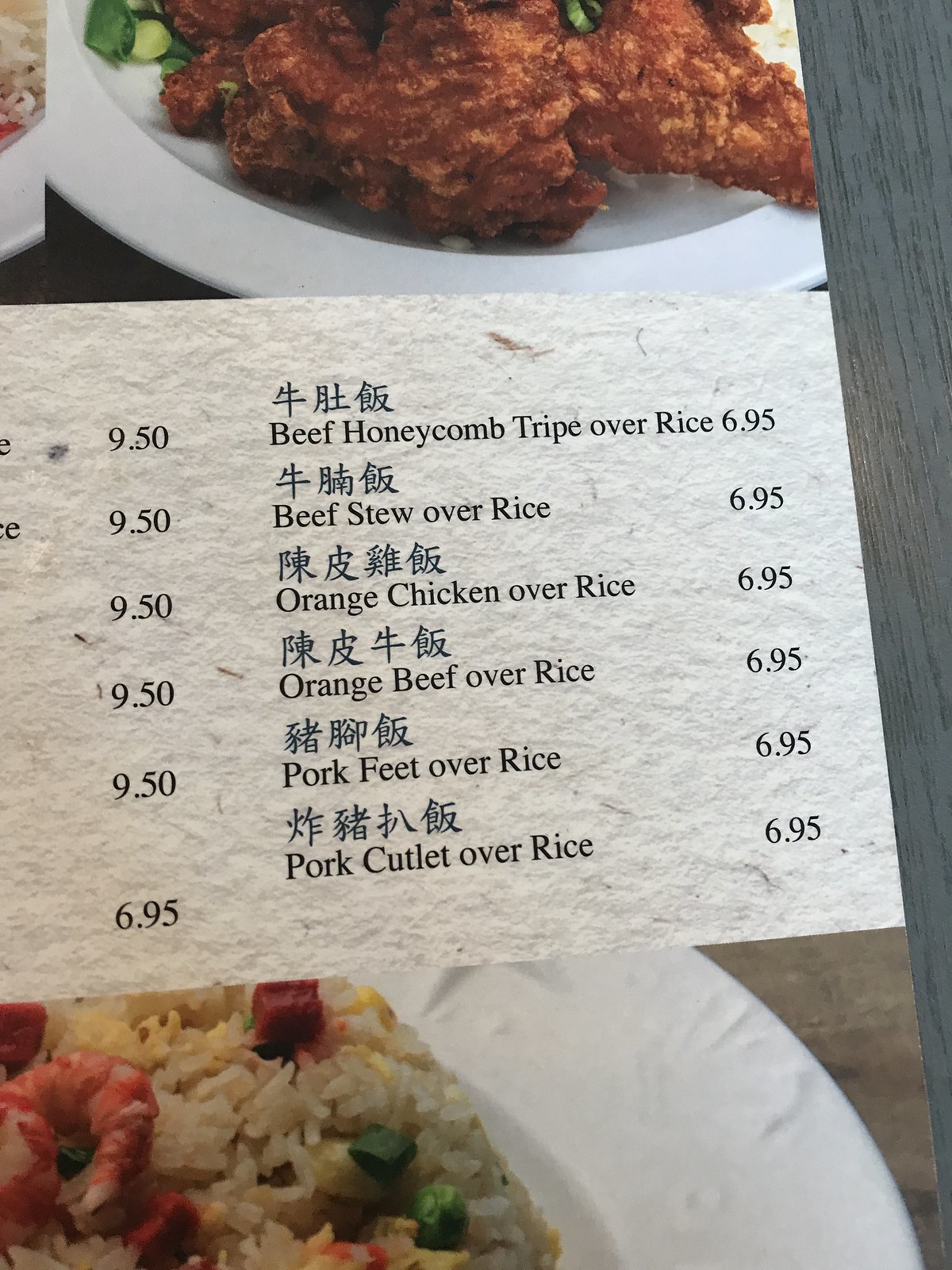The image depicts a partial view of a paper menu from a Chinese restaurant, positioned on a gray painted wooden table. The menu features Chinese characters above the English descriptions of the dishes, all priced at $6.95 on this side of the menu. The visible items include beef honeycomb tripe over rice, beef stew over rice, orange chicken over rice, orange beef over rice, pork feet over rice, and pork cutlet over rice. At the top of the menu is a photograph showing a fried chicken dish garnished with scallions, with an orange hue indicating a likely sauce. Below, another image captures a shrimp fried rice dish on a white plate with visible vegetables such as peas and a single shrimp, sitting on a brown table. Adjacent to this section, an additional portion of the menu is visible, listing several other items priced at $9.50 and one for $6.95. The overall image is slightly grainy and muted in color, with some parts appearing blurred, affecting the clarity of finer details.